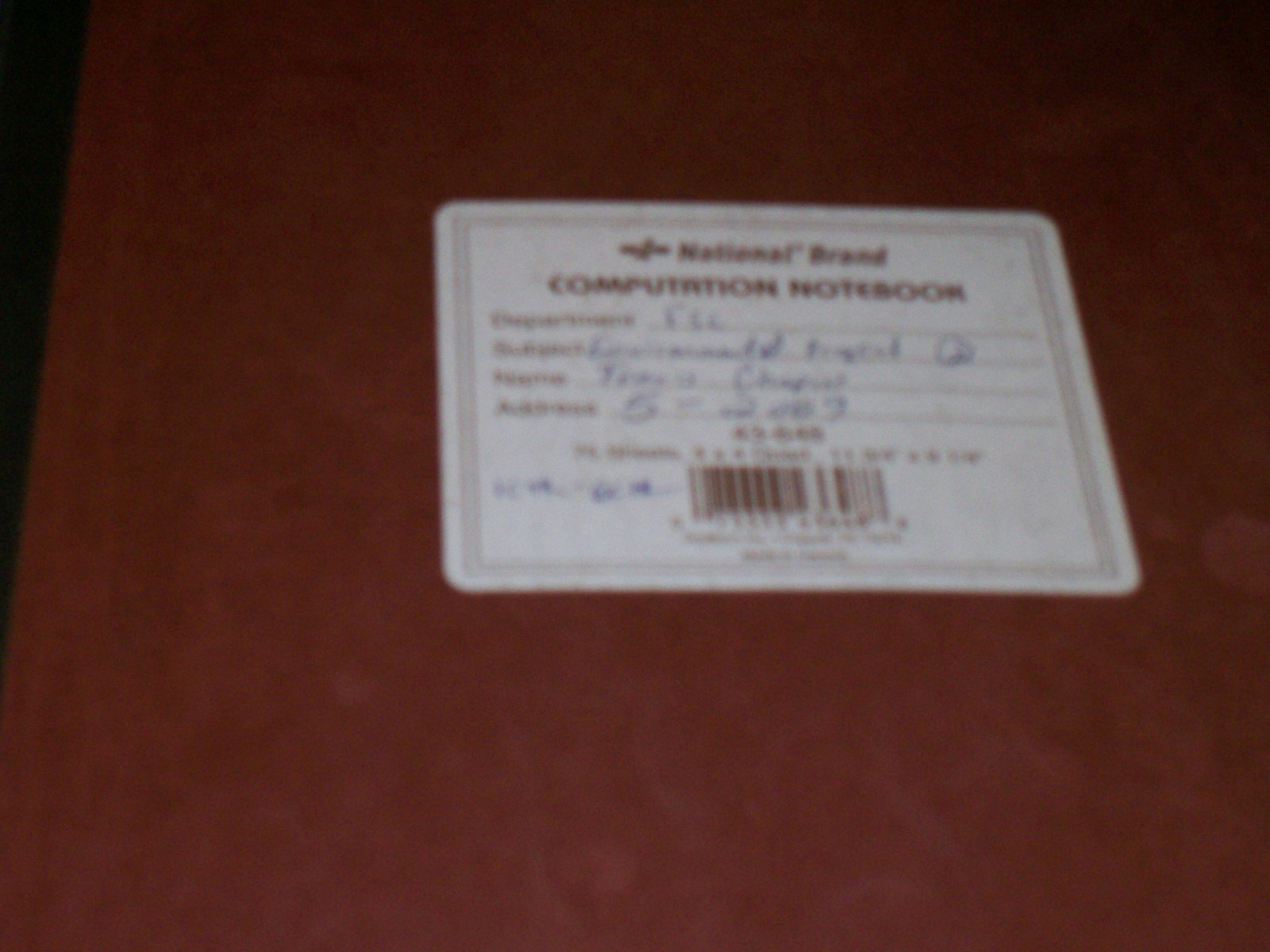The image depicts a blurred photograph of a dark brown notebook, featuring a white, rectangular label with rounded corners affixed to its cover. The label has a straight black border along its edges. At the top of the label, in bold font, it reads "National Brand Computation Notebook." Below the title, there are four distinct fields each accompanied by unreadable text, likely meant for personal information such as name and address, written in blue ink. The bottom of the label displays a barcode. The entire notebook and label are somewhat out of focus, making some details difficult to discern, and there are no people in the photograph. The scene is clearly set against a brown background, either a table or another book.